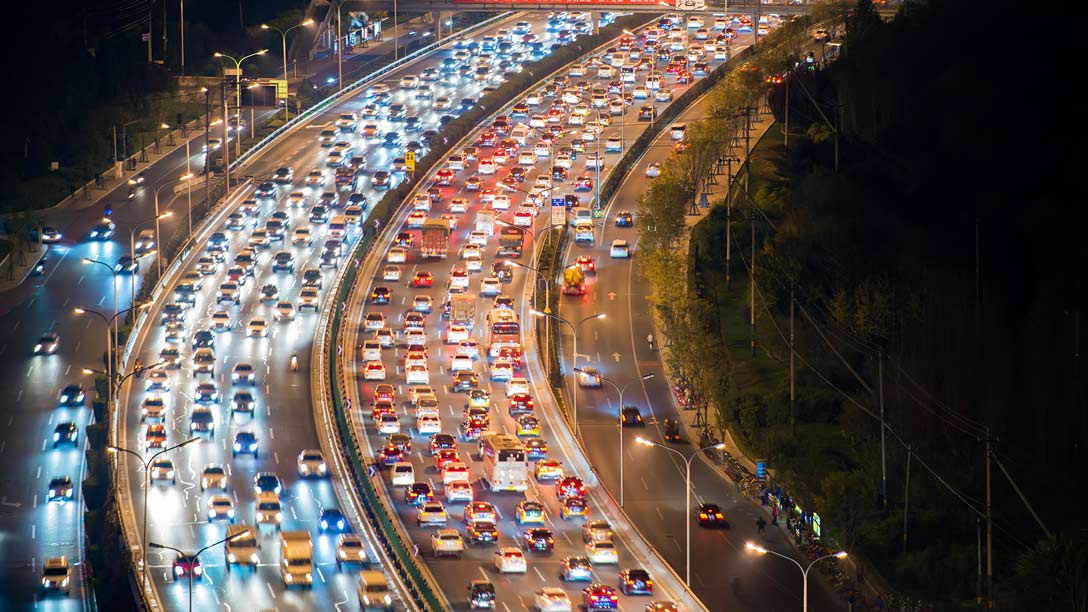This aerial nighttime photograph showcases a bustling freeway system, featuring an elevated eight-lane highway—four lanes in each direction—that is almost entirely bumper-to-bumper with multicolored cars. The freeway, curving from the lower left to the upper right, intersects with other road networks beneath it. There are additional roadways, each approximately three lanes wide, running parallel to the main highway and populated with fewer cars. To the right, the image captures a dark, tree-lined area accompanied by a large metal fence and a ring of electric lines. The photograph is rich in detail, illustrating the intricate flow of traffic with blue headlights visible on cars moving away and red taillights on those approaching. To the left, another road runs in the opposite direction, contributing to the complexity of this crowded urban scene captured from above.